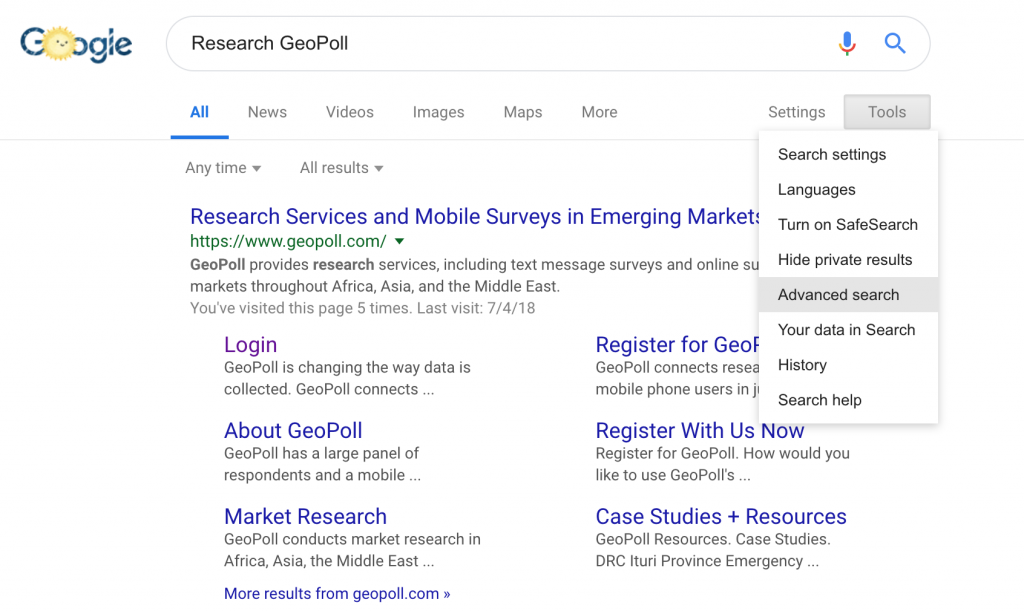A screenshot of a Google search result page captures the special Google Doodle for the day, where the iconic "Google" logo is displayed in blue with white diagonal stripes across it. The first "O" in "Google" has been replaced by a whimsical sun with a simple cartoon face, featuring two dots for eyes and a minimalistic line for a mouth.

At the top of the page, the search bar contains the text "research geopoll". The "All" tab in the menu below the search bar is selected. Adjacent to this menu are two inactive drop-down menus labeled "Any time" and "All results". To the right side, the "Tools" button is activated, revealing a menu with options including "Search settings", "Languages", "Turn SafeSearch on", "Hide Private Results", "Advanced Search" (highlighted in gray), "Your Data in Search", "History", and "Search Help".

The first search result stands prominently in blue text, reading “Research services and mobile surveys in emerging markets." The green URL beneath it is "https://www.geopoll.com", which has an associated drop-down likely meant for viewing cached pages. The description reads, "GeoPoll provides research services, including text messages, surveys, and online", but the rest is obscured by the tools menu. It continues, "markets throughout Africa, Asia, and the Middle East". It also notes that the user has visited this page five times, with the last visit on 7-4-18. 

Further information includes clickable text in purple, "Login" and more details about GeoPoll's services. There are mentions of GeoPoll's significant respondent panel and its focus on mobile market research in Africa, Asia, and the Middle East. The description encourages users to register and explore further with prompts like “case studies,” specific mentions of areas like DRC’s Ituri province, and a concluding link for "more results from geopoll.com".

Overall, the screenshot provides a detailed look at a specific search query, blending visual elements from Google Doodle with informative search results about GeoPoll’s market research services.